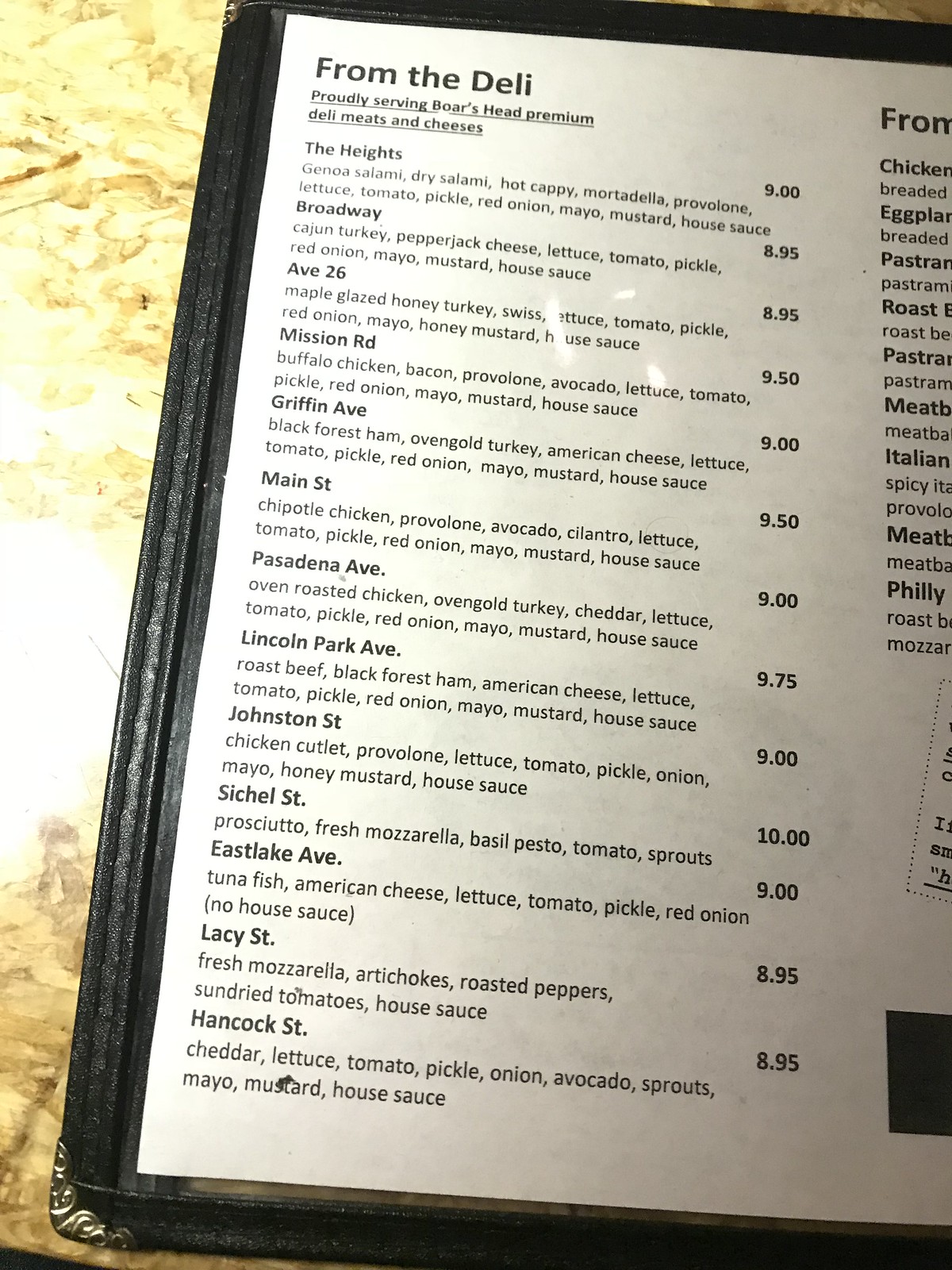This close-up photograph of a menu showcases an array of gourmet sandwiches, each accompanied by their respective prices. The menu is encased in a sleek black leather cover and rests on a countertop featuring a mottled pattern of yellow and brown hues. A bright white glare from the camera's flash can be seen reflecting off the countertop. The menu proudly announces that it serves Boar's Head premium deli meats and cheeses and lists 13 different sandwiches. The first sandwich, aptly named "The Heights," is priced at $9 and includes an assortment of Genoa salami, dry salami, hot cappi, mortadella, provolone, lettuce, tomato, pickle, red onion, mayo, mustard, and a house sauce. Other sandwiches on the menu have equally evocative names such as Broadway, Ave 26, Mission Road, Griffin Ave, Main Street, Pasadena Ave, Lincoln Park Ave, Johnstone Street, Sechelles Street, Eastlake Ave, Lacey Street, and Hancock Street, each detailed with their individual ingredients and costs.